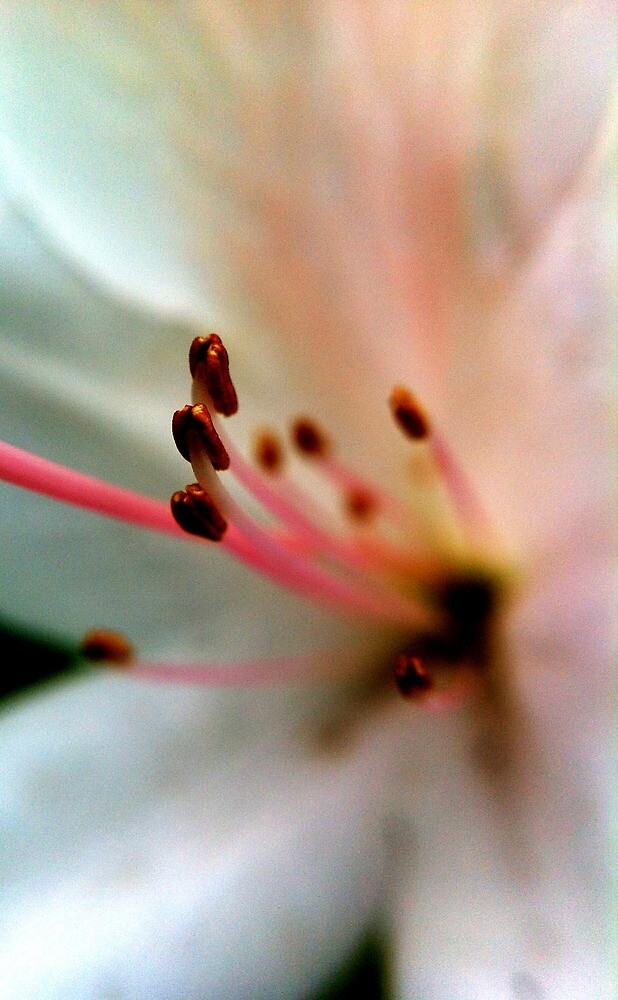This is an incredibly close-up photo of a flower in full bloom, where the focus is primarily on its pistils or stigmas, creating a striking and detailed display. The petals of the flower are predominantly white, with subtle hints of light pink throughout, adding a delicate tint to the overall appearance. These petals form a blurry background for the focal point: the pistils, which protrude conspicuously from the center.

These pistils or stigmas are a distinct pink color and topped with darker, raisin-shaped tips that range in hue from deep brown to reddish. One particularly long pistil extends off-screen to the left, while three others near it are more in focus, progressively getting blurrier as they descend into the flower's core. Additionally, there are several more pistils in varying states of blur, adding to the dynamic composition of the photo.

At the very base of the flower, hints of yellow and black can be discerned, providing additional depth and contrast. Dark green elements in the background suggest an outdoor setting, enriching the natural context of the image. The overall effect is a sharply detailed portrayal of certain parts of the flower, with an emphasis on the intricate and colorful structures within its center.